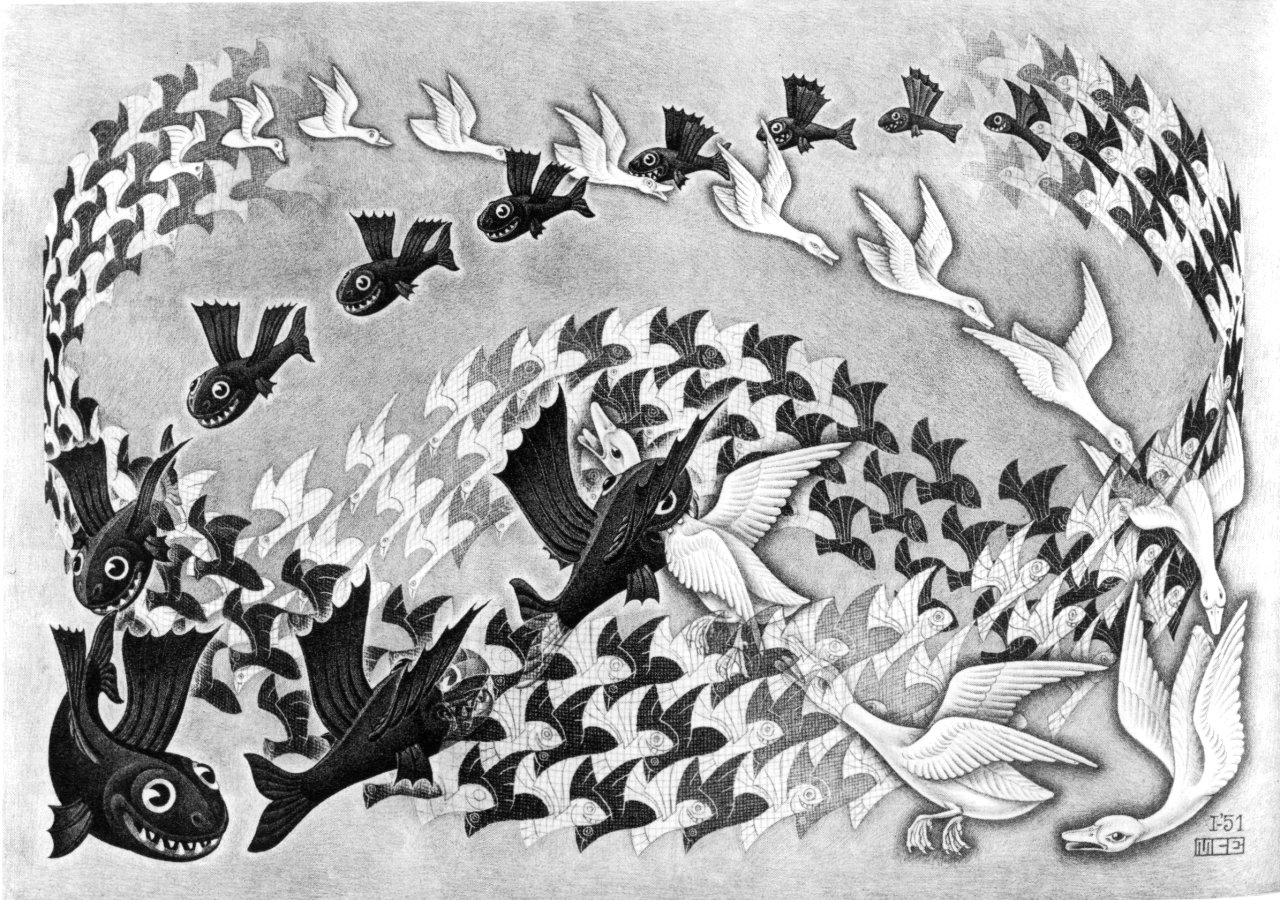This black and white animated design, resembling a sketch or charcoal drawing, intricately depicts black fish with wings and large teeth intertwined with white, dove-like birds. The black fish and the white birds travel in a circular pattern around the picture, with the fish moving counter-clockwise and the birds flying clockwise. This creates a dynamic scene where the two groups meet and cross paths in the center. The design features both small and large repeating images, providing a rich, layered effect. In the middle of the composition, a dramatic focal point is created where a fish bites the neck of one of the birds.